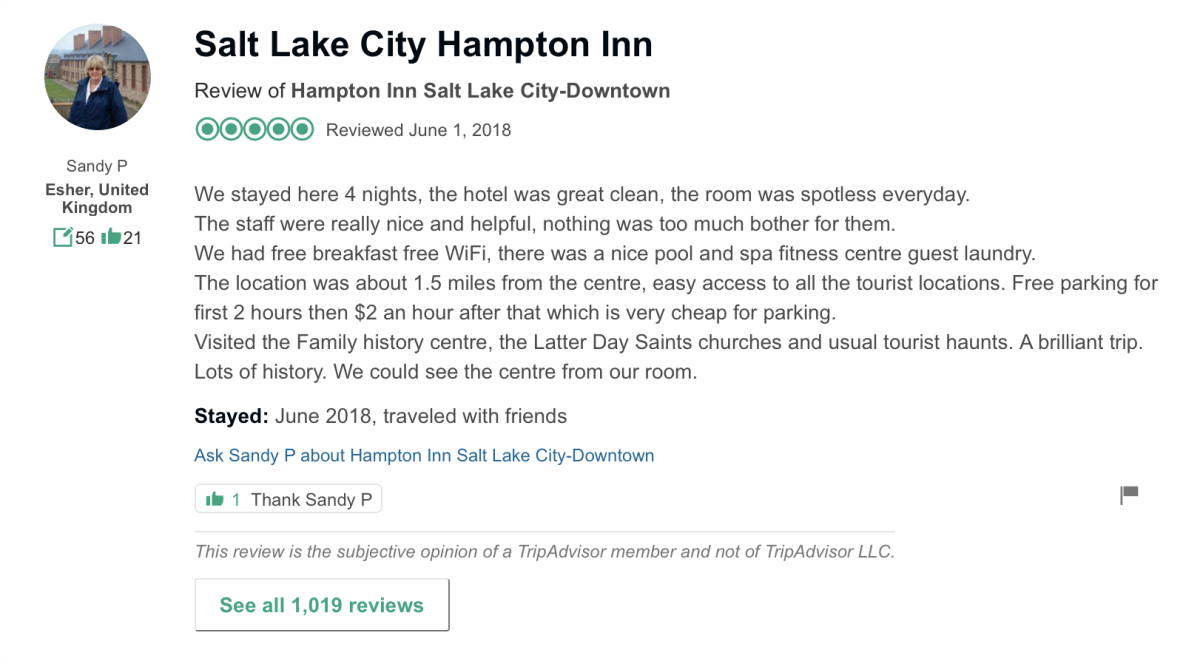**Detailed Caption:**

A screenshot showcasing an online review with a pristine white background and clear black font. In the upper left-hand corner, there is a profile picture of a Caucasian woman, approximately 60 years old, with dyed blonde hair. She is wearing a blue jacket and posing in front of a one-story house. Below her picture, the text reads "Sandy P. Esther, United Kingdom, 56 posts, 21 likes."

Sandy has written a review for the Hampton Inn located in downtown Salt Lake City. Her review, complete with five filled circles indicating a perfect rating, was posted on June 1st, 2018. In her detailed account, Sandy mentions staying at the hotel for four nights and praises the establishment for its cleanliness and helpful staff. She highlights amenities such as free breakfast, free Wi-Fi, a nice pool and spa, a fitness center, and guest laundry facilities. 

Sandy notes that the hotel is located 1.5 miles from the city center, making it conveniently accessible to tourist attractions. The hotel offers free parking for two hours, and then there is a small charge thereafter. During her stay, Sandy visited notable sites including the Family History Center and various Latter-day Saint churches, describing her trip as brilliant and filled with history. She also mentions being able to see the city center from her room.